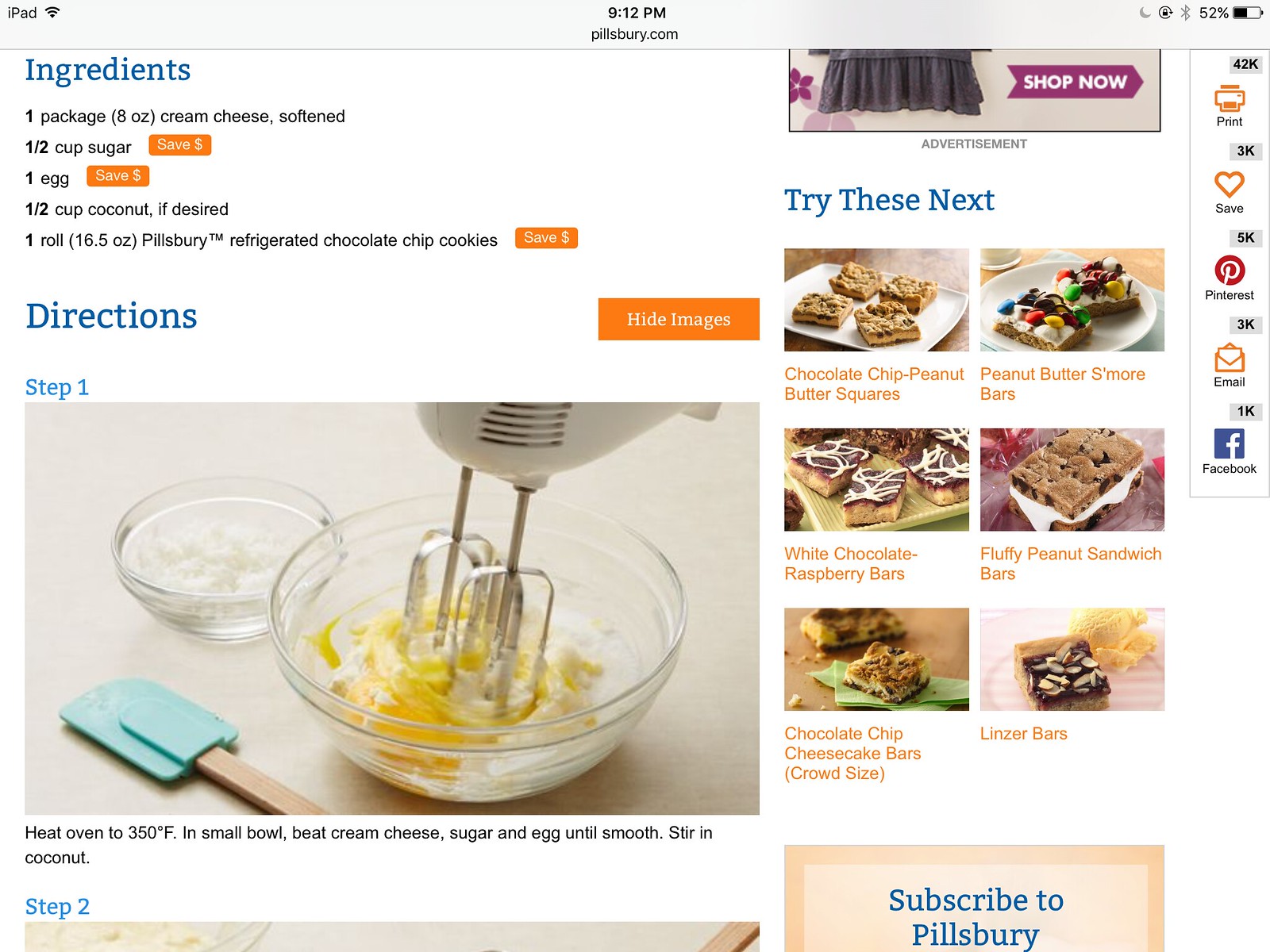This image is a screenshot captured from an iPad at 9:12 p.m., displaying a partially visible recipe from Pillsbury.com. In the top left corner of the screen, next to a Wi-Fi symbol, it reads "iPad." The top right corner shows a battery icon indicating 52% charge, and several other icons for printing, saving, Pinterest, email, and Facebook, each with various interaction counts.

The page details the ingredients and first step for what appears to be a cookie recipe: one 8-ounce package of softened cream cheese, half a cup of sugar, one egg, half a cup of coconut (if desired), and one 16.5-ounce roll of Pillsbury refrigerated chocolate chip cookie dough. The image associated with step one displays an electric mixer beating the ingredients in a bowl, with a rubber spatula and a small clear cup, presumably containing water, nearby. Step one instructs to preheat the oven to 350°F, and to beat the cream cheese, sugar, and egg until smooth before stirring in the coconut.

On the right side of the screen, there is a "Try These Next" section featuring six other baking recipes, including chocolate chip peanut butter squares, peanut butter s'more bars, white chocolate raspberry bars, fluffy peanut sandwich bars, chocolate chip cheesecake bars (labelled for a crowd size), and Linzer bars. Each recipe is accompanied by a small photograph. The bottom of the visible page includes an invitation to subscribe to Pillsbury in blue letters on a tan background.

The overall layout is user-friendly, with ingredient lists and directions clearly written in blue headers, and vibrant images enhancing the visual appeal of the page. The screenshot provides a detailed glimpse into a digital baking recipe experience on an iPad.